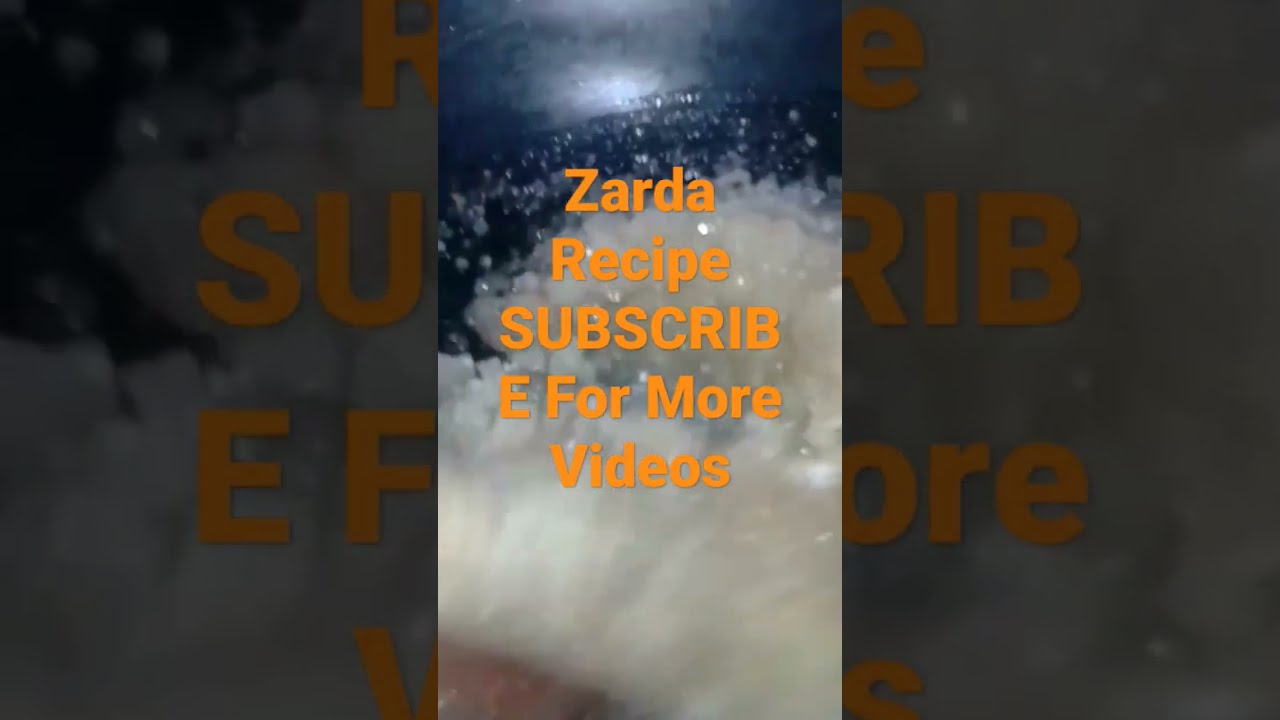This is a pixelated screenshot, possibly from a YouTube or TikTok video, in portrait orientation, taken at night. The image features a crowd of people in the background with white foam or bubbles being dumped on them. The foreground prominently displays this white foam. Overlaid on this chaotic scene is a black pot or bowl, potentially containing sautéed onions or a similar glistening, mushy, white substance. Superimposed across the image in bold orange sans-serif font are the words "Zarda Recipe. Subscribe for more videos," where the last letter of "subscribe" is cut off and placed on a new line. The "E" is in capital letters, making "subscribe" appear as "subscrib" with the "E" on the next line. The caption suggests this is a promotional image enticing viewers to subscribe for more culinary content.